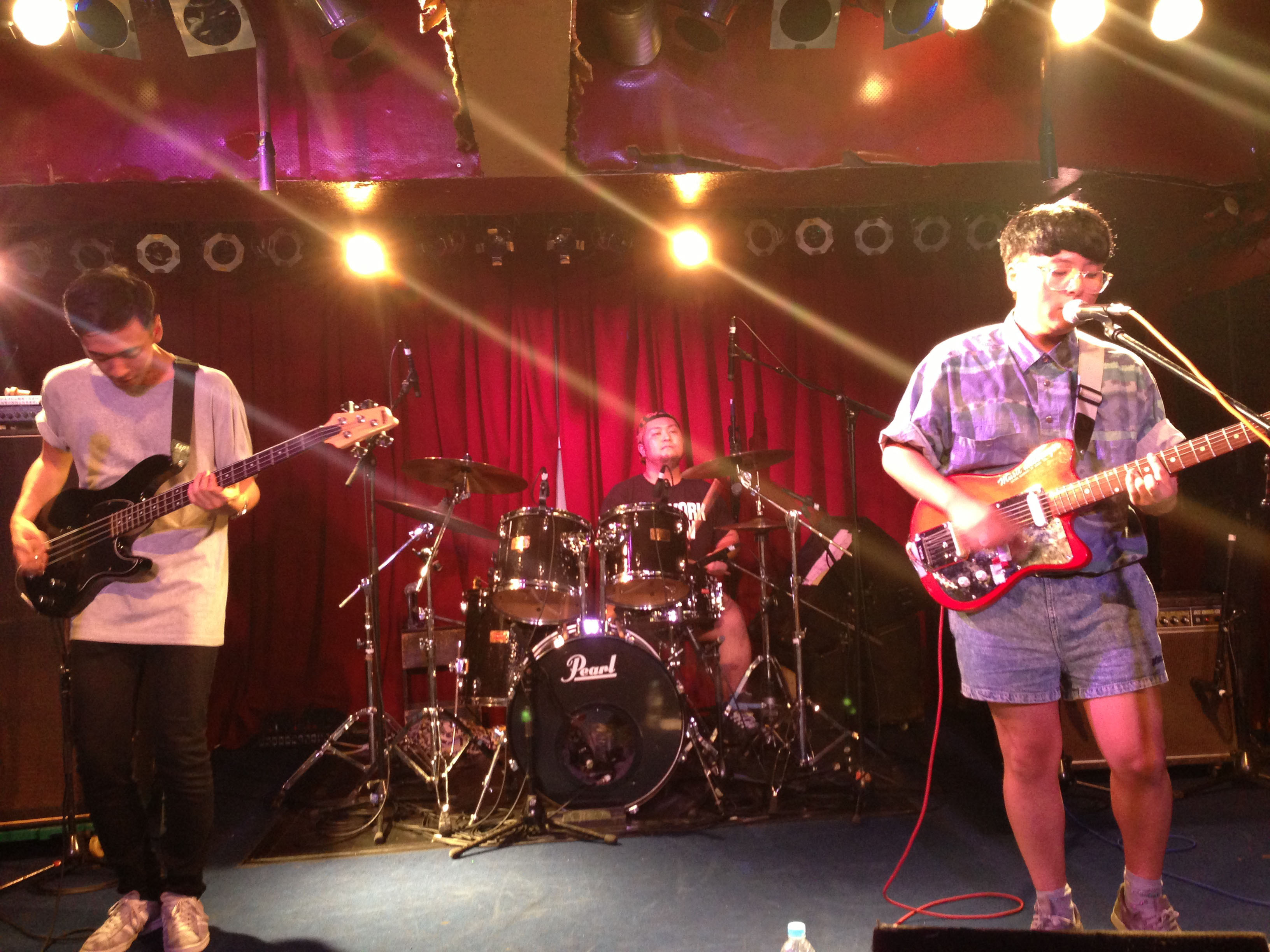In this photo, an Asian band is captured in the midst of a performance on a small stage, surrounded by dynamic strobe lights and a red curtain as a backdrop. The lead singer, positioned on the right, is a young man with brown hair, glasses, and a black bowl haircut. He is dressed in jean shorts, sneakers, and a light blue plaid shirt, passionately singing into a microphone while playing a red electric guitar. To his left stands the bassist, who is adorned in black pants, sneakers, and a white T-shirt. He has black hair and is intently focused on his black electric guitar. Centrally located behind a large black drum set is the drummer, identified by his black T-shirt and khaki shorts, energetically keeping the rhythm. The gray-colored floor beneath them contrasts with the vibrant lights above, illuminating the scene. Although the audience is not visible due to the close-up nature of the photo, the presence of stage equipment and lighting suggests a sizable venue for their performance.